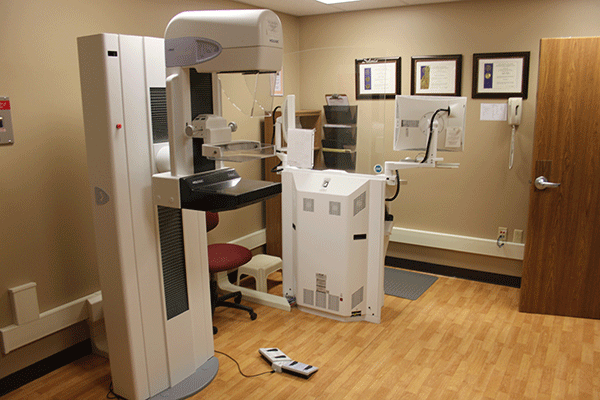Inside a doctor's office with beige-colored walls and wood-paneled floors, the room features an array of medical equipment and furnishings. On the left side, there is a large, white machine that occupies a significant portion of the space. This device has a platform at the bottom and appears to have clear and black shelves, possibly suggesting an x-ray machine setup. Adjacent to this is a red chair, and nearby, a cable runs across the floor. 

In the corner of the room, a smaller machine incorporates a computer with a visible display screen. This setup is mounted on a white rectangular structure. Above and near this equipment, three framed plaques or certificates decorate the wall, along with a yellowish landline phone positioned below one of these frames. A black filing cabinet with a clipboard rests beside the frames. 

A mysterious device on the ground resembles a foot pedal, though its specific function is unclear. The door to the room is open, allowing easy access. This detailed arrangement provides a comprehensive view of a well-equipped medical office, blending clinical functionality with professional decor.